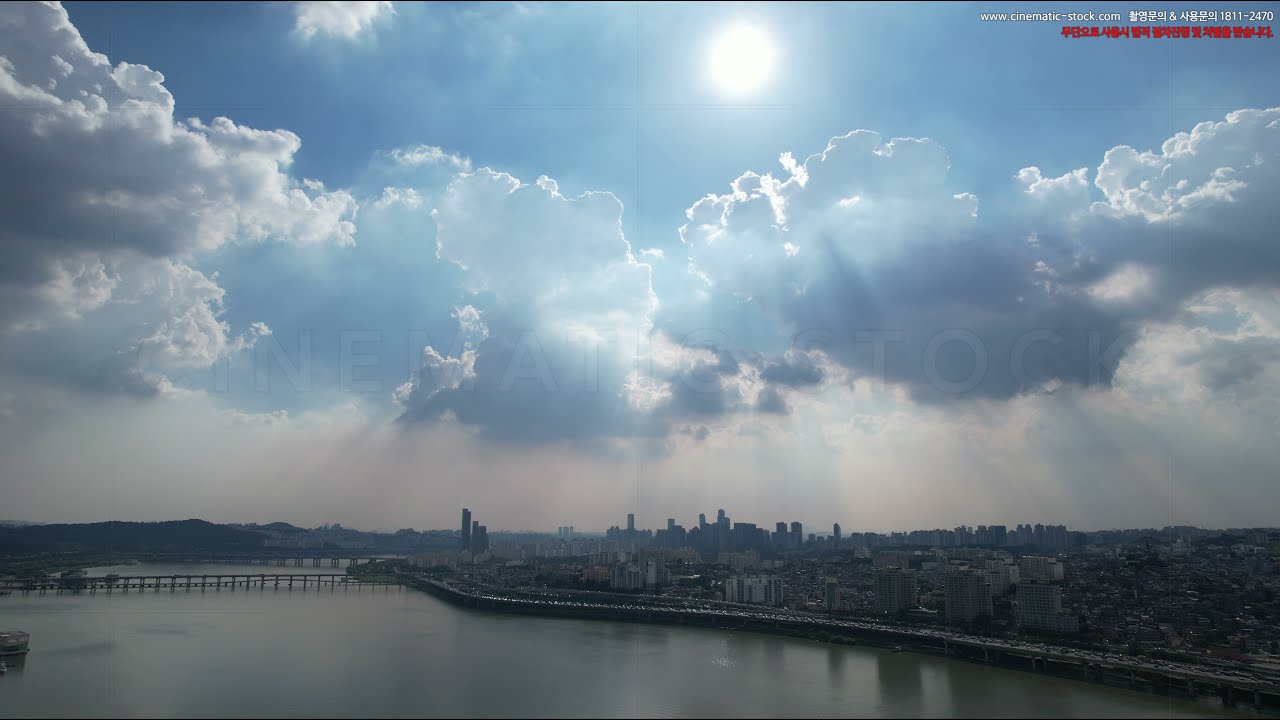A professionally captured, mid-overhead shot of a large city skyline is set against a light blue sky adorned with various white and gray clouds. The top center of the image features the sun peeking through the cloud cover, casting a natural light over the cityscape below. Dominated by an array of towering skyscrapers and smaller buildings, the city extends toward the horizon. In the bottom left corner of the image, a greenish-gray river, still and reflective, winds its way close to the urban area, flanked by distant hills. A prominent bridge spans the river from left to right, facilitating the flow of traffic towards the bustling city. Between the river and the city lays a large, busy highway teeming with cars traveling in both directions. This image captures the dynamic and intricate interplay of natural and urban elements, framed perfectly by the sky and clouds above.